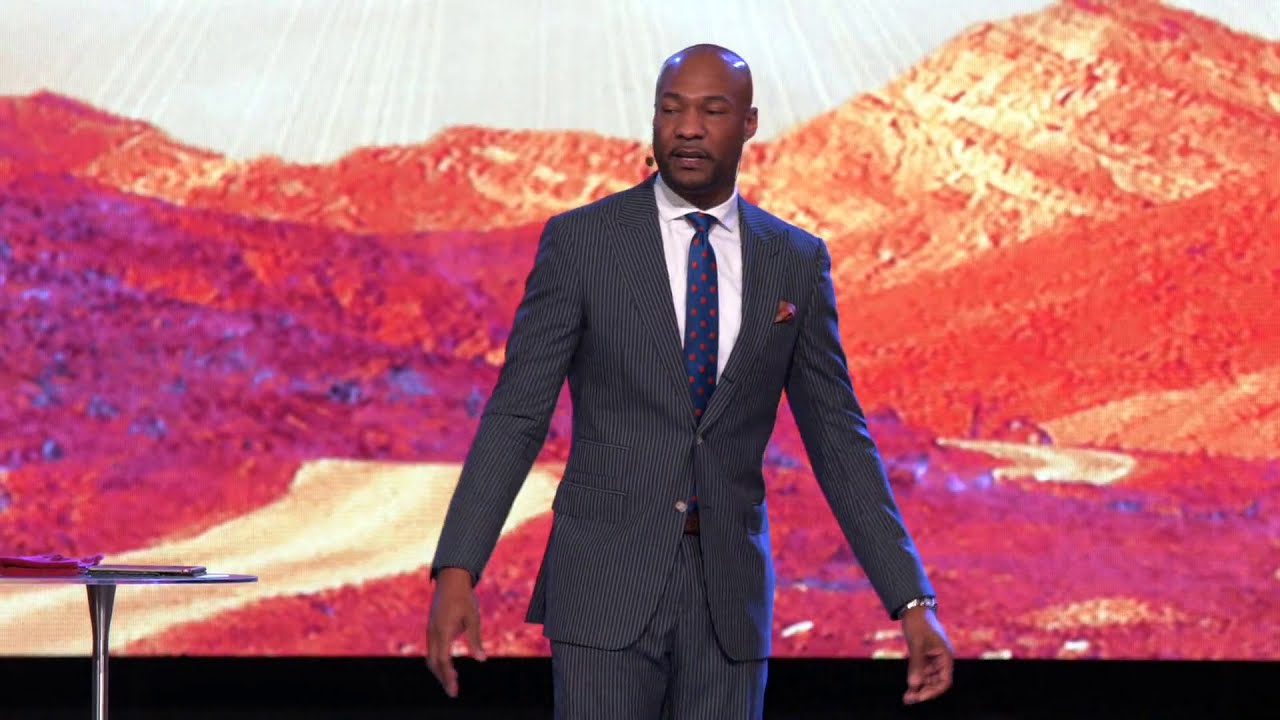A distinguished bald black man stands confidently with his eyes closed, arms slightly outstretched from his hips, dressed in an elegant and tailored gray pinstripe suit. His suit jacket, which has one button undone, is paired with a pristine white shirt and a blue tie adorned with red speckles. A red handkerchief neatly peeks out from his suit pocket, complementing his meticulous appearance. He wears matching striped slacks, and a gold watch or bracelet on his right wrist adds a touch of sophistication. The light reflects off his bald head, highlighting his poised demeanor, accentuated by a slight mustache. A minimalistic metal table with a glass top stands to his left, accompanied by an electronic device, possibly an iPad. Behind him, a background featuring vivid blue, orange, and yellow paint formations contrasts strikingly with the projected image of scenic, sandy mountains, dotted with sagebrush and magenta floral elements, giving a Southern California vibe. Blue lighting from the right side further enhances his professional stage presence, hinting that he might be addressing an audience, perhaps in a role such as a preacher, indicated by the tiny microphone on his left ear.